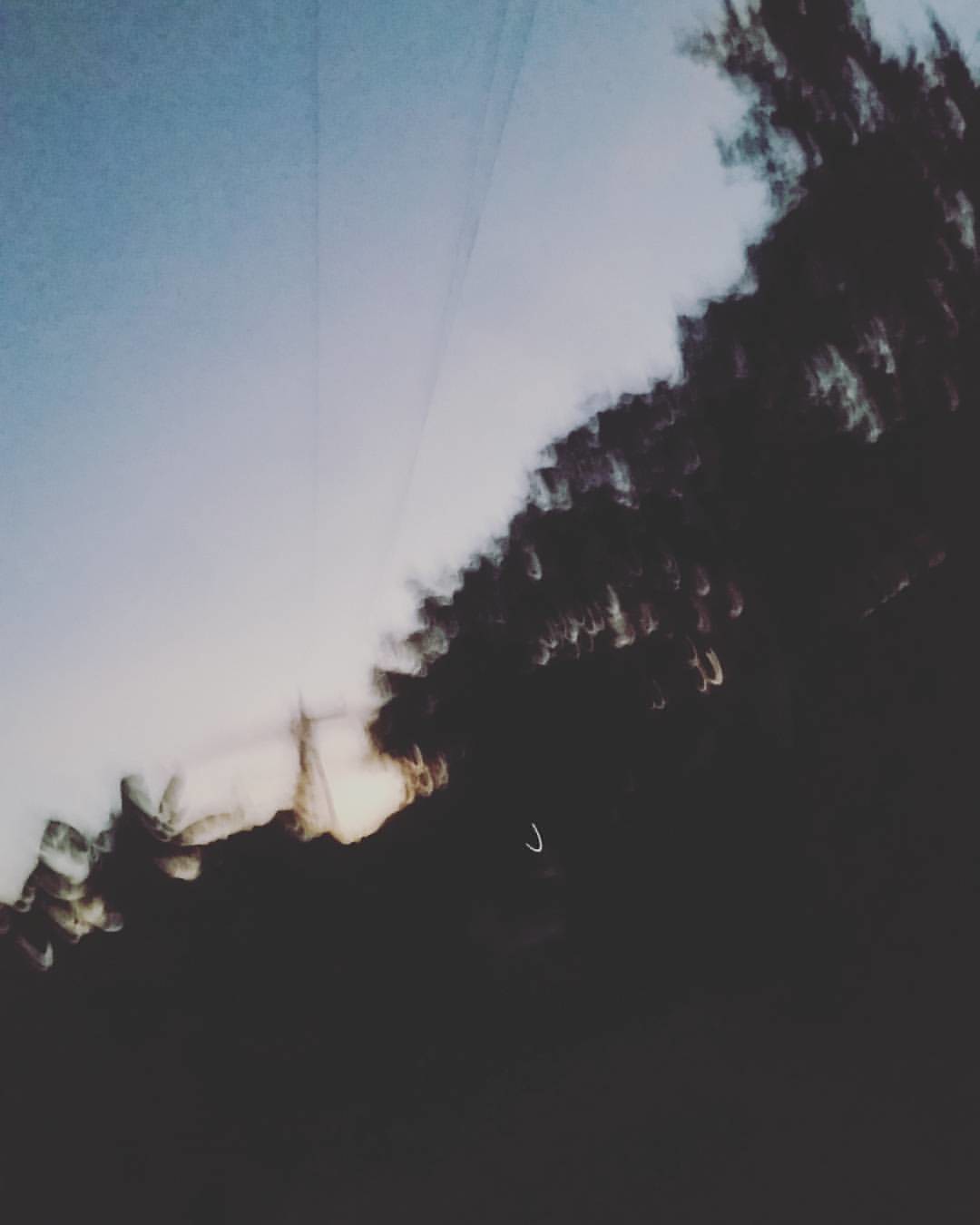The photograph captures a shadowy, silhouetted forest scene during either sunrise or sunset, with the sun low on the horizon, bedimming the details of the surroundings. Tree silhouettes form a dark border against a gradient sky transitioning from deep blue to the remaining light of the sun. The image, taken from ground level and directed upwards, reveals power lines cutting across the top portion of the frame, emphasizing an everyday intersection of nature and man-made structures. The scene is blurry, with no flash used, giving it a dreamy, almost abstract quality. The overall effect is a striking contrast between the dark foliage and the dimly lit sky, capturing the serene and transitional time of dusk.